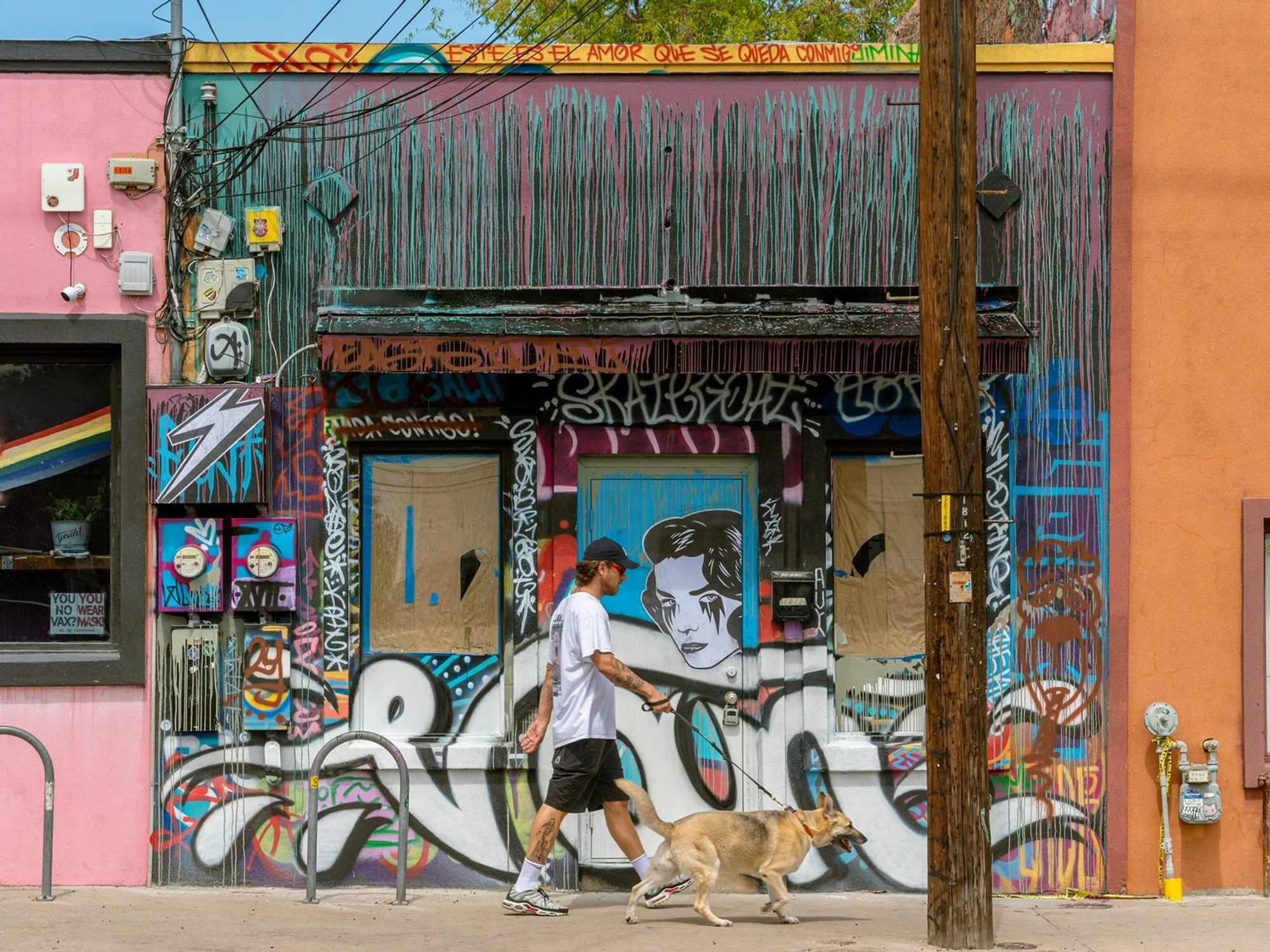In this horizontal rectangular image, a man is walking his large, light brown German Shepherd with dark brown spots on a sidewalk, in front of a colorful, graffiti-covered storefront. The man, moving from left to right, wears a white t-shirt with something on the back, black shorts, tube socks, athletic white shoes, a black hat, and red sunglasses. He sports a tattoo on his leg and one on his forearm, holding a black leash. The storefront behind them, likely closed with boarded-up windows, features various graffiti art, including a woman's face with dark hair and running mascara, a white octopus with a head, and an array of blues, whites, and pinks on what seems to be a once-black facade. To the left, the pink building's wall is partially covered by spillover graffiti, and a small rainbow adorns its window. To the right, the neighboring building is orange. The scene captures a small slice of blue sky and green foliage, while a prominent wooden telephone pole stands in the foreground on the sidewalk.